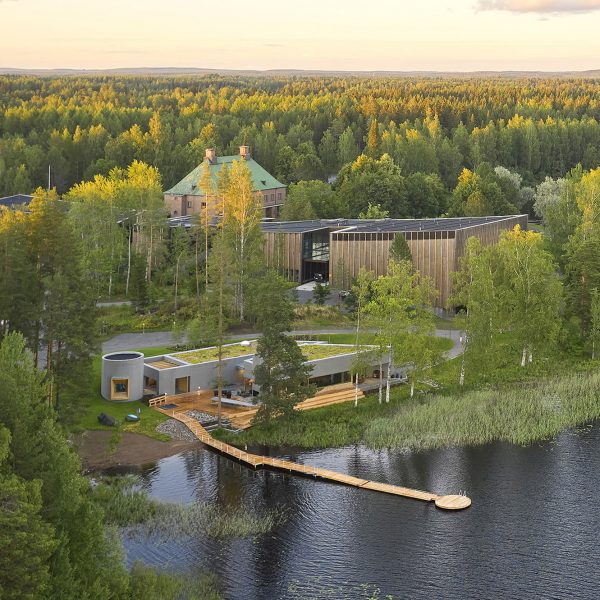This overhead drone image captures a picturesque lakeside scene dominated by a flat-roofed house with a small cylindrical tower on its left side and a deck on the front. This house, surrounded by lush green grass and bordered by dense trees, sits near the shore of a tranquil lake. A wooden pathway extends from the left side of the house and leads to a dock that stretches out into the water, where a small boat is moored.

To the right of the house, a winding gray driveway curves around, eventually exiting the image to the left. Beyond this driveway is a large industrial building, possibly a manufacturing facility, and another large building with a green roof and two chimneys. The backdrop of the scene is a vast, dense wooded area with rolling hills on the horizon. The entire scene is bathed in the soft, pale hues of a peach-toned sky with a solitary cloud in the upper right corner, adding a serene ambiance to this idyllic landscape.